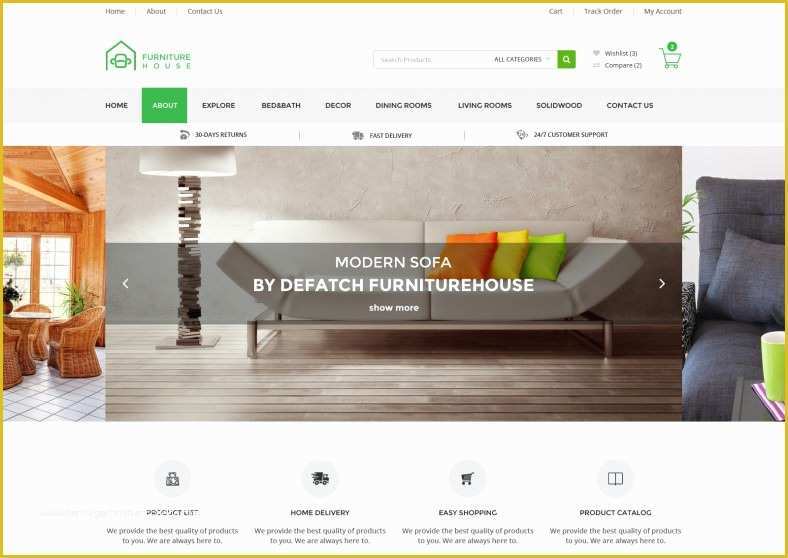The image depicts a website dedicated to selling furniture, prominently branded as "Furniture House" in the upper left corner. Above the name, a navigation menu features links to "Home," "About," and "Contact Us." On the upper right, the options "Cart," "Track Orders," and "My Account" are listed. Below this main navigation, there is a search bar that includes a dropdown menu labeled "All Categories" and a search icon, which is white on a green square background.

Adjacent to the search bar, the site displays a "Wishlist" with three items and a "Comparison List" feature, seemingly holding three items as well. Further down, another navigation menu offers links to various sections: "Home," "About," "Explore," "Bed and Bath," "Decor," "Dining Rooms," "Living Rooms," "Solid Wood," and "Contact Us."

Promotional features below this navigation include "30 Days Return," "Fast Delivery," and "24-7 Customer Support." The center of the page showcases a high-quality photograph of a modern couch, described as a "Modern Sofa by D. Fatch Furniture House," with a "Show More" link and a right arrow for further exploration. 

Flanking this central image are partial views of additional photographs that are part of a carousel, inviting users to scroll through more options. Directly below, the page highlights sections titled "Product List," "Home Delivery," "Easy Shopping," and "Product Catalog." The entire website design is framed by a distinctive yellow outline.